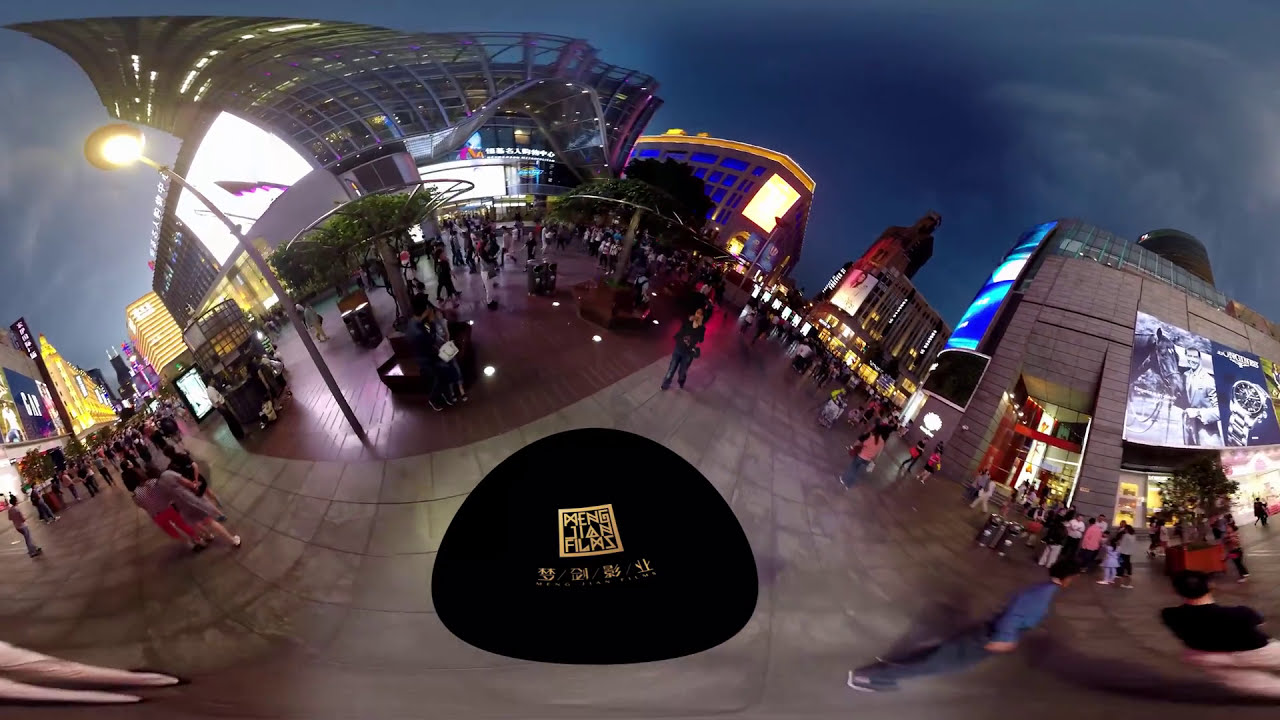This is a highly detailed, nighttime panorama of a bustling city street, potentially in Tokyo, featuring distorted optical lens effects that give it a rounded, somewhat warped appearance. The concrete sidewalk is laid out in a crisscross pattern of square blocks, contributing to an illusion of unevenness across a seemingly flat surface. The scene is illuminated by an array of bright lights, making the dark blue sky almost secondary to the vibrant shopping area bustling with activity.

On the left side of the image, various stores are visible, including a prominent GAP store marked by its recognizable navy blue square with white capital letters. Nearby, other stores are lit with yellow and purple lights, enhancing the lively atmosphere. The right side features additional stores adorned with numerous billboards and neon signs, emphasizing this area's commercial nature. 

In the center, there seems to be a communal indoor-outdoor patio area, with trees and other natural elements like hanging baskets of grass, possibly serving as a food pavilion or rest area. This central spot stands out with a circle in the black concrete, hinting at a potential logo for a film company, suggesting a theater might be nearby. People are seen leisurely wandering, shopping, and congregating, underscoring the area as a vibrant, well-maintained, and busy night-life hub.